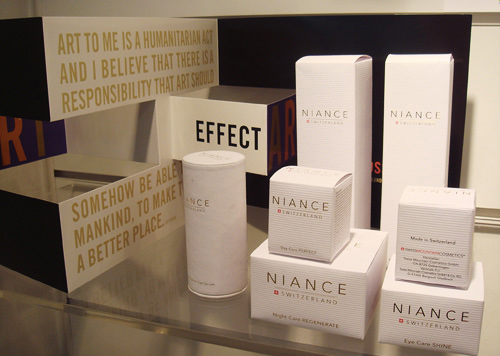The photograph depicts an angled display case showcasing a variety of Niance beauty product boxes. The display is arranged on a clear, tiered shelf. Each product is packaged in pristine white boxes featuring black lettering, and prominently includes the Niance brand name followed by "Switzerland" with the Swiss flag symbol in red and white beside it. There are various box shapes: tall and rectangular, square, and one cylindrical container, all neatly positioned. Among the visible labels, one box reads "Night Care Regenerate," while another says "I Care Perfect," and others are marked with product names like "I Care Shine." Additionally, a decorative text on the side of the display reads: "Art to me is a humanitarian act. I believe that there is a responsibility that art should somehow be able to affect mankind to make a better place."